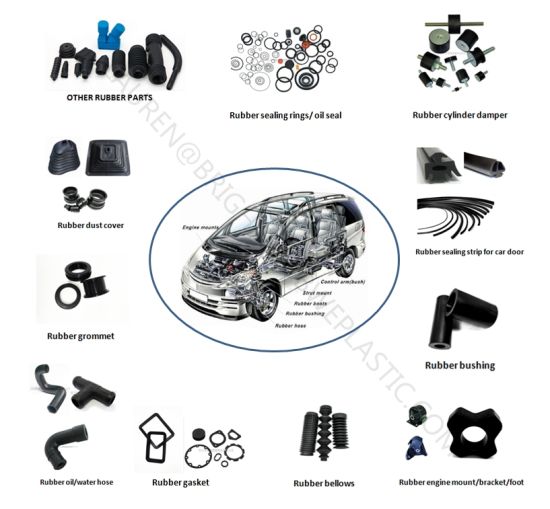The image is a detailed diagram of various car parts, centered around a cutaway drawing of a minivan that provides a see-through view of its internal components, including the engine, seats, wiring, chassis, and wheels, all surrounded by an oval. Surrounding the central van image are multiple labeled illustrations of different rubber car parts. At the upper left section, there are blue and black rubber parts labeled "Other Rubber Parts." To the top right, black circles are labeled "Rubber Sealing Rings/O-Seal," while adjacent to it another section is labeled "Rubber Cylinder Damper." On the lower level of the image, there are black parts labeled "Rubber Desk Cover." The diagram also includes labels for additional parts such as rubber bushings, grommets, gaskets, and bellows, all necessary for car manufacturing. The background features faint, unreadable watermarking, suggesting it's from a website specializing in these rubber components.